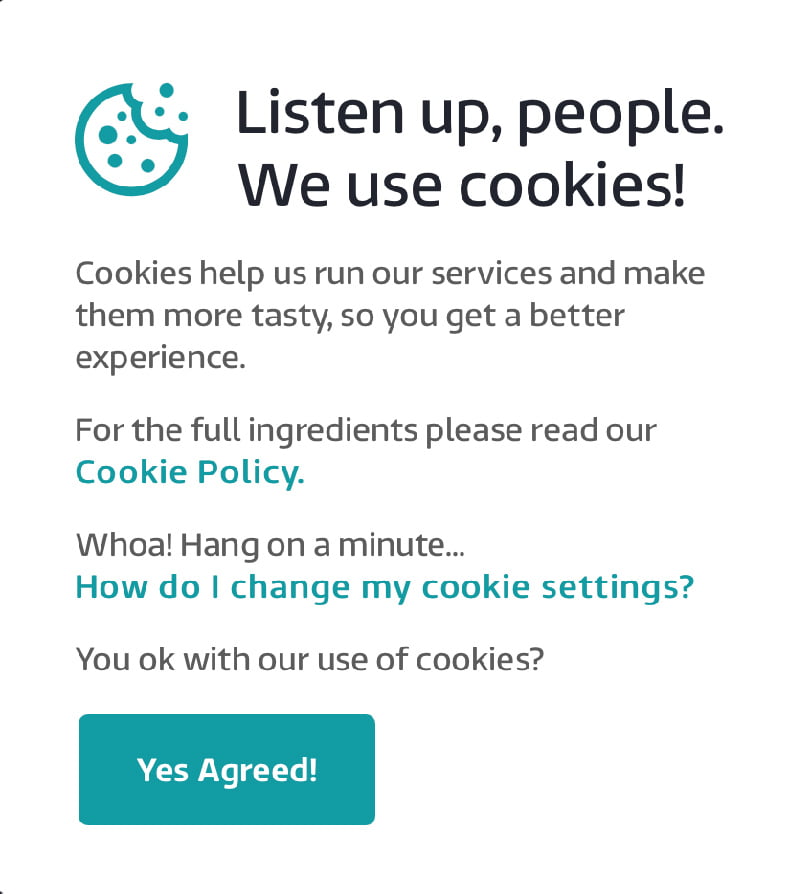This image appears to be a smartphone screenshot depicting a cookie policy notification from a website. On the left side, there is a logo of a bitten cookie. To the right, in bold black text, it reads "Listen up, people. We use cookies!" Below this, in gray text, the notification continues: "Cookies help us run our services and make them more tasty so you get a better experience. For the full ingredients, please read our cookie policy." The message then poses a question followed by an ellipsis, asking, "How do I change my cookie settings?" Lastly, there is a bolded question in black text: "You OK with our use of cookies?" Beneath this question is a prominent green button with white text that says "Yes, agreed!" This notification serves to inform users about the website's use of cookies to enhance user experience and guides them to additional information and settings.